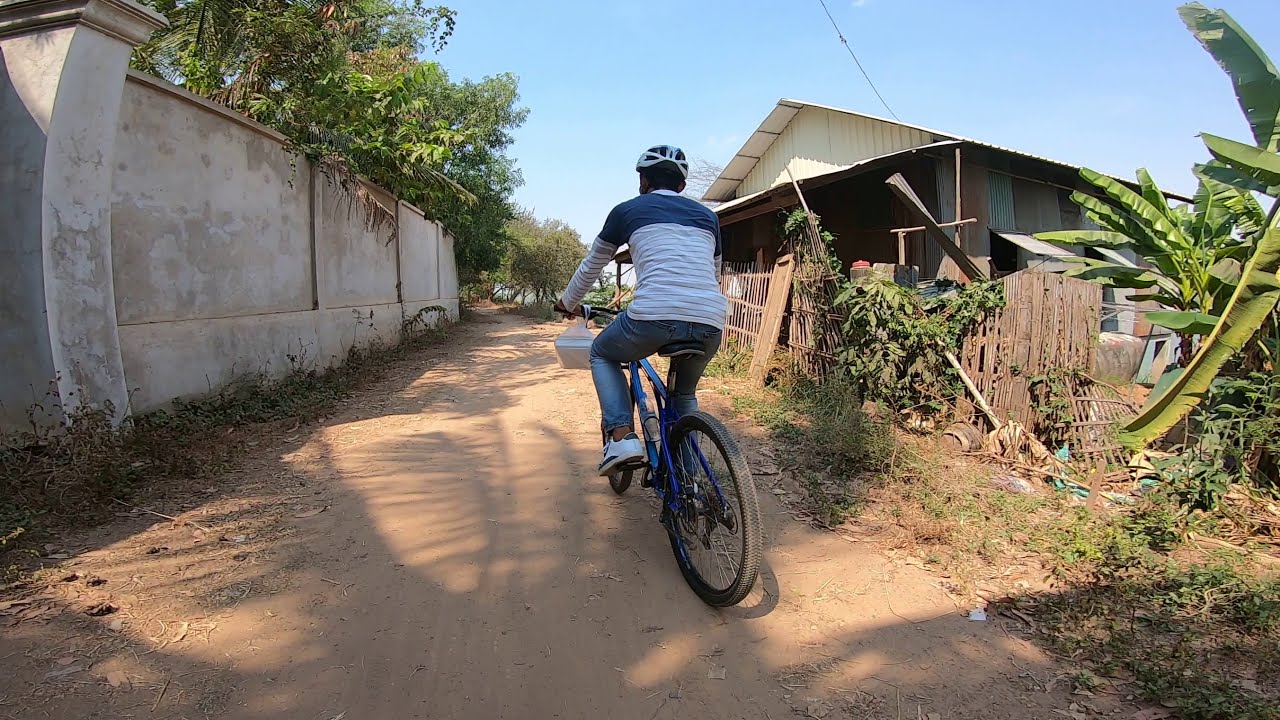The image captures a scene on a wide dirt road, flanked by various structures and greenery. A man, dressed in blue jeans, white trainers, and a long-sleeved shirt with dark blue shoulders and thin blue stripes, rides a dark blue bicycle. He is also wearing a white bicycle helmet. Attached to the left handlebar of his bike is a plastic bag containing a box, suggesting he might be delivering something. 

On the left side of the road stands a tall concrete wall with peeling plaster and low shrubbery at its base. Overhanging the wall are some trees, adding to the greenery. To the right, there is a partially collapsed old brown wooden fence and a shed-like structure made of sheet metal and wood, topped with a white tin roof. The area also features some low leafy trees and palm-like plants peeking into the scene.

The pathway recedes into the distance, lined with both living and dead plants, and opens up to more trees far ahead. The sky is a clear light blue, indicating daytime with no visible clouds.